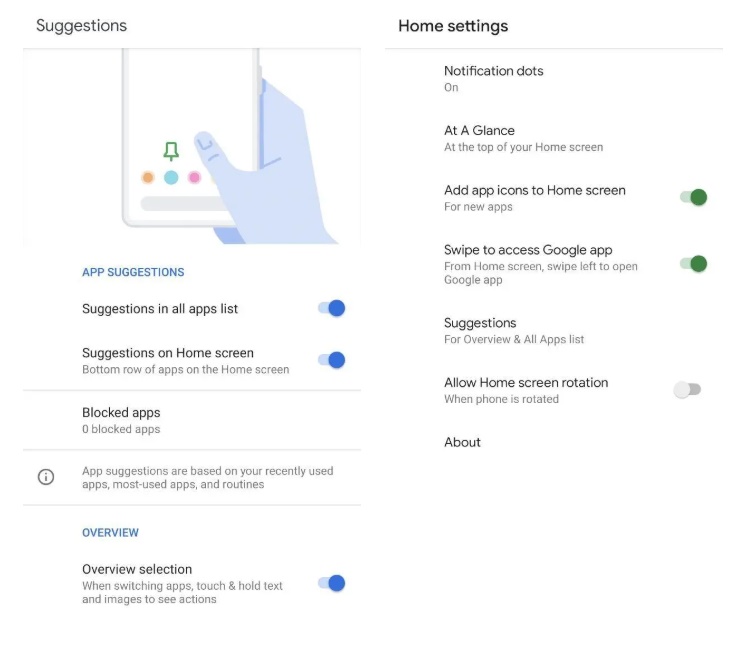This image is a screenshot of a webpage or phone interface displaying settings and options for app and home screen management. 

On the left side, there is a "Suggestions" section. This section includes various toggles such as "Suggestions in all apps list" and "Suggestions on home screen," both of which have the button turned blue, indicating they are enabled. There is also a note about "Blocked apps" showing zero blocked apps. Further details explain that app suggestions are based on recently used apps, most used apps, and routines. Below this, blue text reads "Overview," followed by black text stating "Overview selection." It explains that when switching apps, you can touch and hold text and images to see actions, with a blue button to the right of this explanation.

On the right side, there is a "Home settings" section. This section lists various options including "Notification dots" and "At a glance at the top of your home screen," both of which appear to be enabled. Additional options such as "Add app icons to home screen," indicated with a green button selected for new apps, and "Swipe to access Google app," which also has a green toggle for swiping left from the home screen to open the Google app, are shown. Completing this section, options for "Suggestions," "Allow home screen rotation," and "About" are listed.

The background of the interface is predominantly white with the majority of the text in black, providing a clean and simple visual layout.